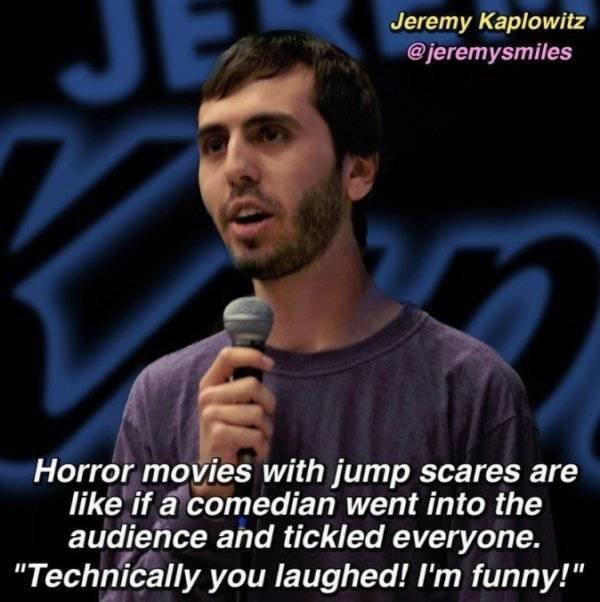In this photograph, there is a white man, presumably a comedian, with short dark brown hair and a stubbly beard and mustache, holding a microphone up to his mouth. He is wearing a long sleeve gray shirt. The background is black with blue lettering that is somewhat blurred, and it appears to say "Jeremy" in the background. In the top right corner of the image, it states in yellow text, "Jeremy Kaplowitz," and underneath that in white text, "@Jeremy Smiles." Superimposed at the bottom of the image in white text is a quote from his standup act: "Horror movies with jump scares are like if a comedian went into the audience and tickled everyone. Technically you laughed, I'm funny." The man appears to be facing the audience, mouth open, as if in the middle of delivering a joke. His eyes are very dark and he has smooth, clear skin. The neon blue outlines in the background add a vibrant contrast to the otherwise dark setting.